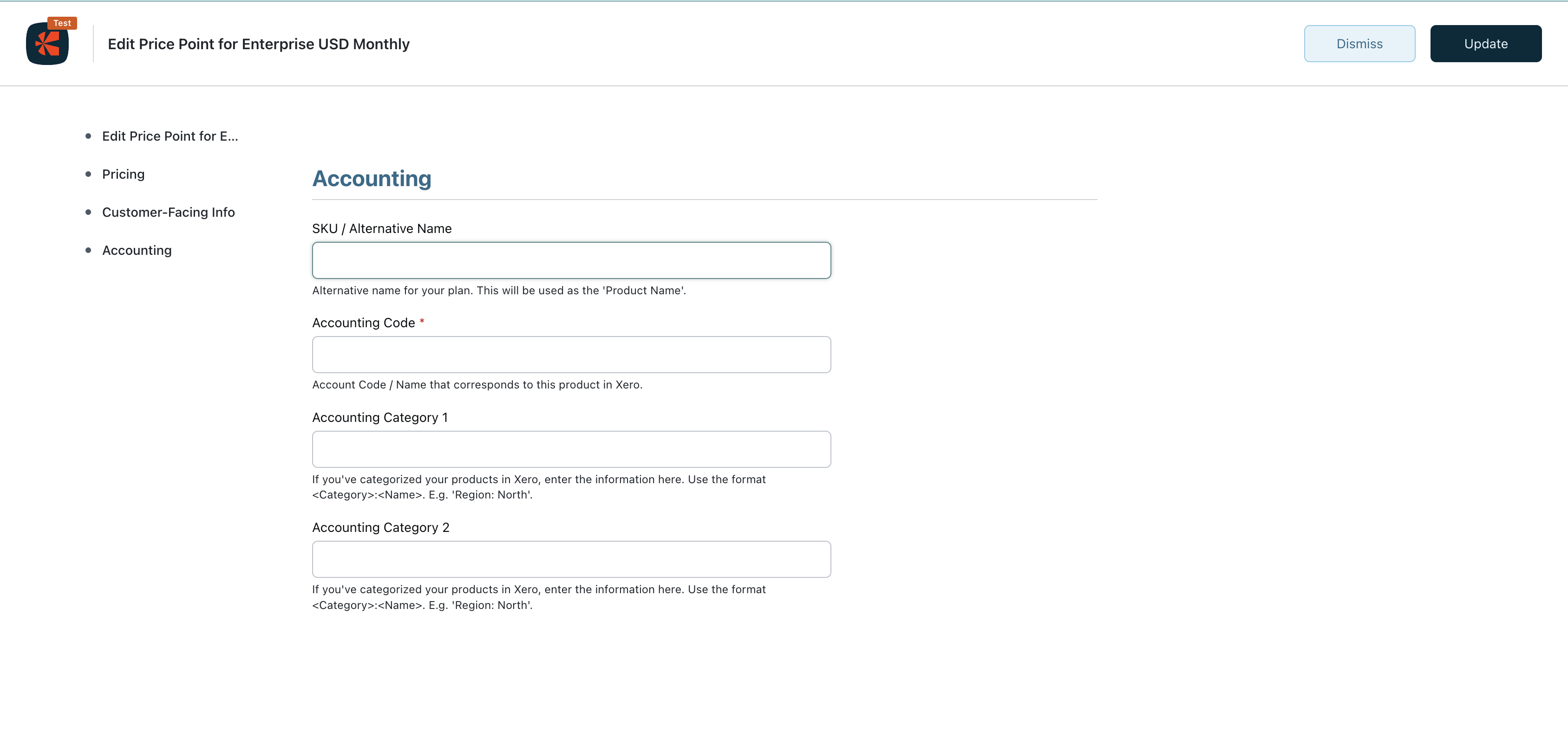The image depicts a detailed section of an enterprise pricing configuration interface for a monthly USD subscription. On the left side, there is a prominent icon resembling a red flower set against a blue background, with an orange label that reads "test" on a white field.

Alongside the icon, there is a list of four bullet points:
1. Edit price point for e-pricing
2. Customer-facing info
3. Accounting
4. (Details of the fourth point are not provided)

The current section highlighted is "Accounting." This section includes various fields for inputting and editing financial information related to the product:

- "SKU/Alternative Name": This field is empty and prompts the user to enter an alternative name for the plan, which will be used as the product name.
- "Account Code/Name": Also empty, this field asks for an account code or name that corresponds to this product in the Xero accounting software.
- "Accounting Category 1": An empty data field with a note underneath instructing users to enter product categorization information in a specified format (e.g., "category: name.region: region: nor") if their products are categorized in Xero.
- "Accounting Category 2": Another empty data field with similar instructions for entering categorization data for the product in Xero.

The interface is designed to allow precise customization and detailed financial tracking for enterprise-level products.